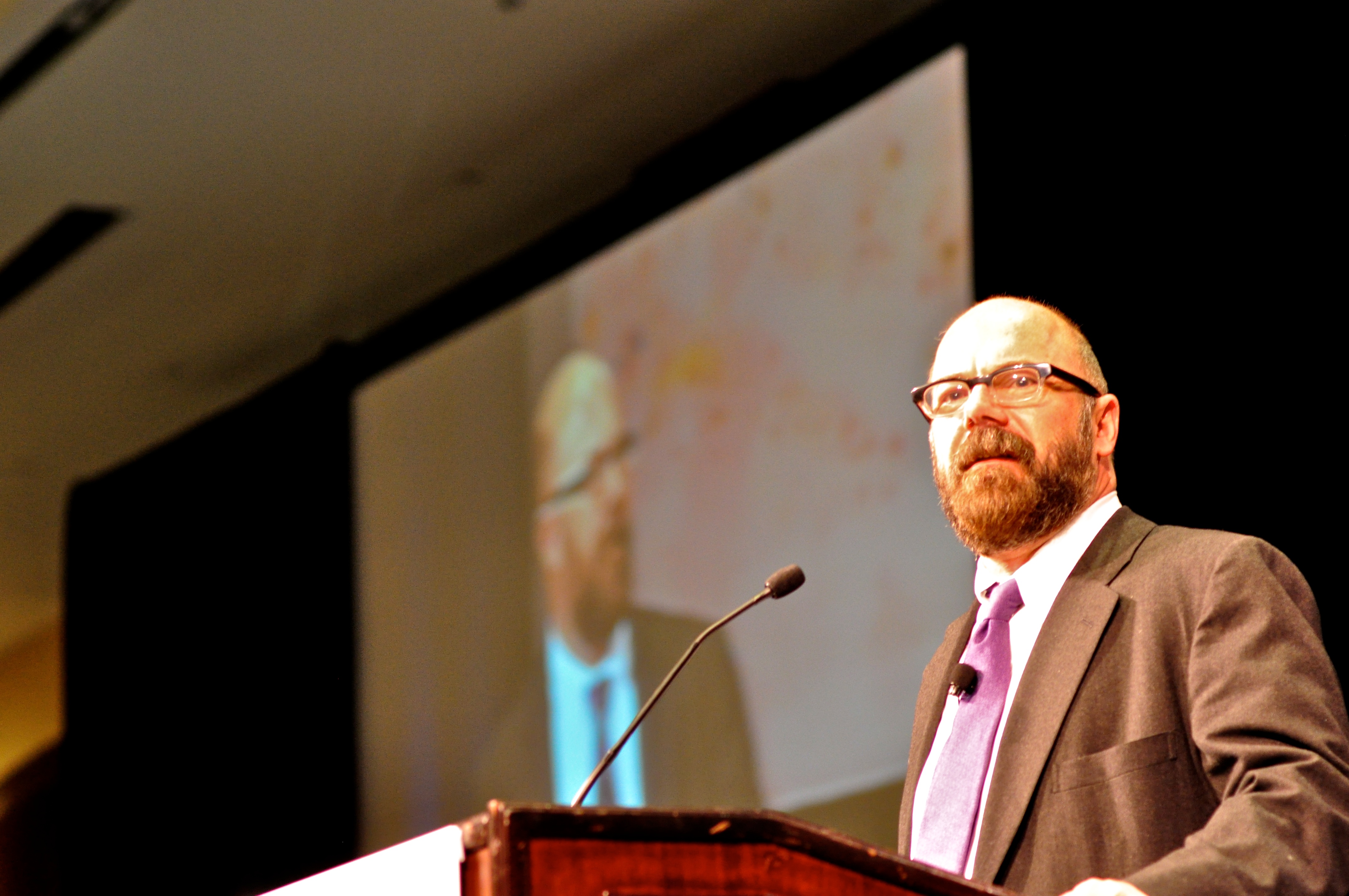In this detailed image, a man, who is white, stands at a podium speaking into a microphone. He is dressed in an ill-fitting dark brown or gray jacket, accompanied by a white shirt and a notably colorful tie that blends hues of pink and purple. He also sports a somewhat long, reddish-brown beard and is wearing glasses. His balding hair is cropped closely to his head. A black microphone is clipped to his tie, emphasizing his preparedness for the speech.

The setting is a brightly lit auditorium, with a contrasting dark stage backdrop consisting of a large black curtain. The podium itself is crafted from a brownish-reddish wood, partially adorned with a white draped fabric that adds a formal touch. Positioned behind him is a projection screen displaying his image from another angle, making it seem as though the audience can see him up close despite the vastness of the space. Interestingly, the projected image of his suit appears darker. The screen also features a background with a mottled pattern of white, pink, and orange, possibly resembling an abstract painting. This combination of live and projected visuals creates a dynamic scene, with the well-lit figure of the speaker standing against the darker, yet detailed, backdrop.